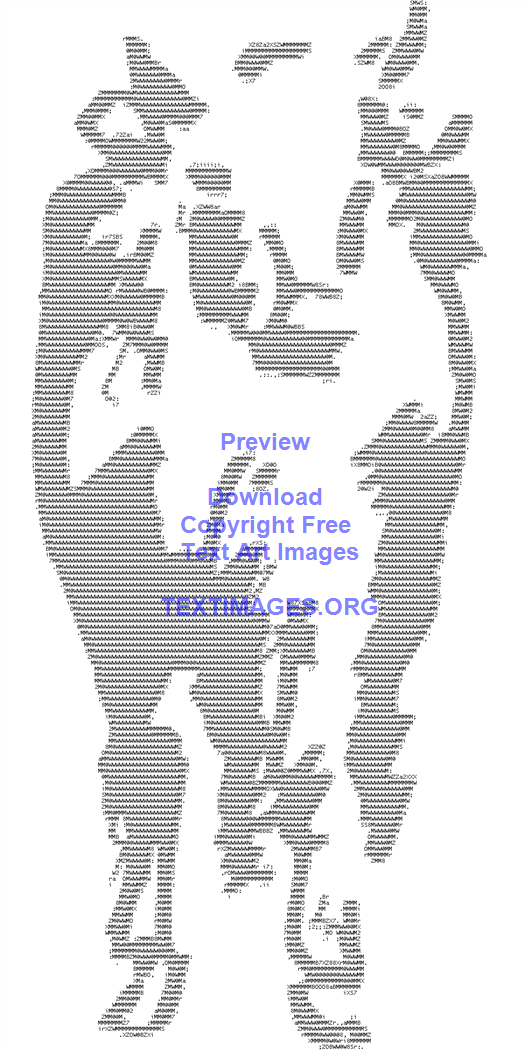This digital image features a stylized black-and-white depiction of a bull, meticulously crafted using the repeated letter "M" to form an intricate text art design. The artwork is predominantly white with the bull's outline and details, such as hooves and horns, defined through the dense, black text. At first glance, the intricacy of the text can make the bull's form challenging to discern, but stepping back reveals the full complexity of the creature, reminiscent of a pointillist technique. Centrally positioned within the image in light purple text, a message reads: "preview, download, copyright-free text art images," followed by "TEXTIMAGES.ORG" in all caps. This indicates that the artwork originates from textimages.org, where users can presumably download it without the watermark. This unique blend of text and digital artistry creates a compelling visual experience that emphasizes both the craft of text art and the striking image of the bull.